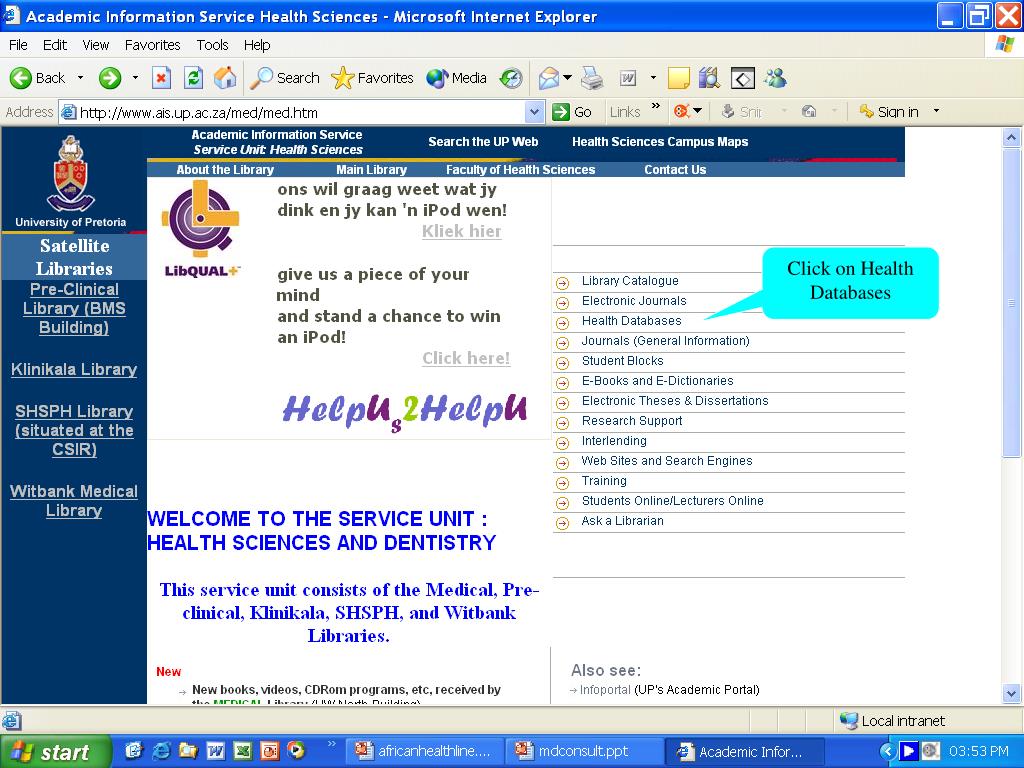**Descriptive Caption:**

This screenshot showcases the web page for the Academic Information Service Health Sciences, as viewed in Microsoft Internet Explorer. Dominating the left side of the page is a vertical blue banner, featuring a shield icon at the top adorned in red, gold, and blue. Beneath the shield, the text reads: "University of Pretoria, Satellite Libraries, Preclinical Library, BMS Building, Clinical Library, SHSPH Library, situated at the CSIR, and Witbank Medical Library."

The upper section of the webpage spans horizontally with navigational options including "Academic Information Service," "Service Unit Health Sciences," "Search the UP Web," and "Health Sciences Campus Maps." Directly below this header, additional clickable sections are titled "About the Library," "Main Library," "Faculty of Health Sciences," and "Contact Us."

On the right side of the webpage, a prominent blue speech bubble highlights a key interactive feature, guiding users to "click on Health Databases." This pointer directs attention to a comprehensive list located in the main content area, which includes "Library Catalog, Electronic Journals, Health Databases, Journals, General Information, Student Blocks, E-books and E-dictionaries, Electronic Theses and Dissertations, Research Support, Interlending, Websites and Web Engines, Training, Students Online/Lecturers Online, and Ask a Librarian."